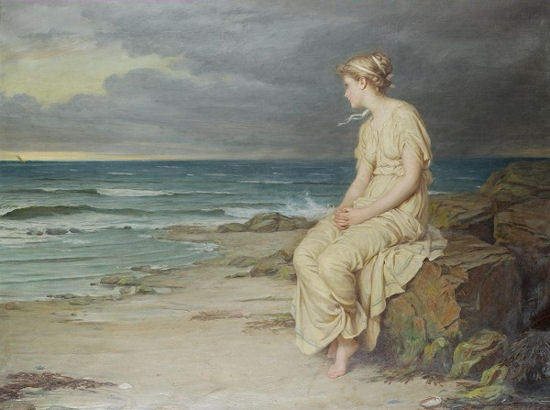In this somber and muted painting, a woman sits alone to the right of the frame on a collection of brown and green, rusty, jagged rocks at the beach. She wears a long, cream-colored dress and has her pale feet and arms bare. Her hair, a blend of blonde and brown, is tied up in a bun adorned with a ribbon. Facing left, her gaze is directed towards the endless, blue-gray ocean where white ripples and small waves crash gently. The sandy shore is a mix of tan and brown hues, dotted with dark spots indicating moist areas. Above her, a predominantly dark and purplish sky, heavy with storm clouds, dominates the scene, though some pale sky peeks through the upper left corner. The air is thick with a sense of approaching dusk as the color palette deepens, capturing the tranquil yet melancholic essence of an overcast day by the sea. The water appears to be inching closer to her feet, emphasizing her solitude amidst the vastness of nature.